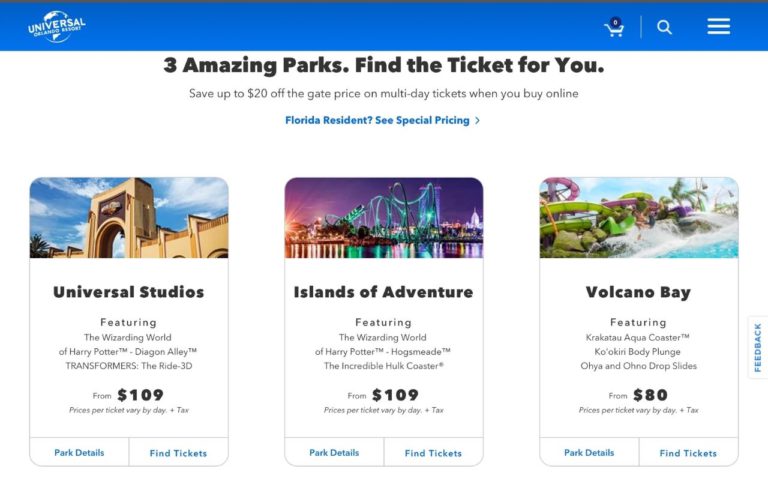The advertisement for Universal Studios prominently showcases their official website's layout, featuring a distinct blue navigation bar across the top. On the left side of the bar, the Universal Orlando Resort logo is prominently displayed, signaling the brand. Moving to the right side of the bar, there's an embedded shopping cart icon, a magnifying glass for search, and a three-line menu icon for additional site navigation options.

Beneath this navigation bar, the center of the ad highlights in bold text, "Three Amazing Parks. Find the Ticket for You." Just below this, there's a special offer that reads, "Save up to $20 off the gate price on multi-day tickets when you book online." Additionally, there's a note for Florida residents about special pricing.

The main body of the advertisement is divided into three sections, each promoting a different Universal Studios park with corresponding images and details:

1. **Universal Studios Entrance**: This image features the grand entrance to Universal Studios, emphasizing popular attractions like The Wizarding World of Harry Potter, Diagon Alley, and Transformers: The Ride 3D. The ticket price is listed as starting from $109. At the bottom, there are links for park details and ticket purchasing options.

2. **Islands of Adventure**: The centerpiece image shows this park illuminated in the evening, creating a magical and adventurous atmosphere. The starting price for tickets is also $109.

3. **Volcano Bay**: The final image showcases one of the thrilling rides at Volcano Bay water park, with ticket prices beginning at $80.

Overall, this detailed and visually appealing advertisement effectively conveys the excitement and value of planning a visit to Universal Studios' trio of parks, while providing clear information on how to secure discounted tickets.